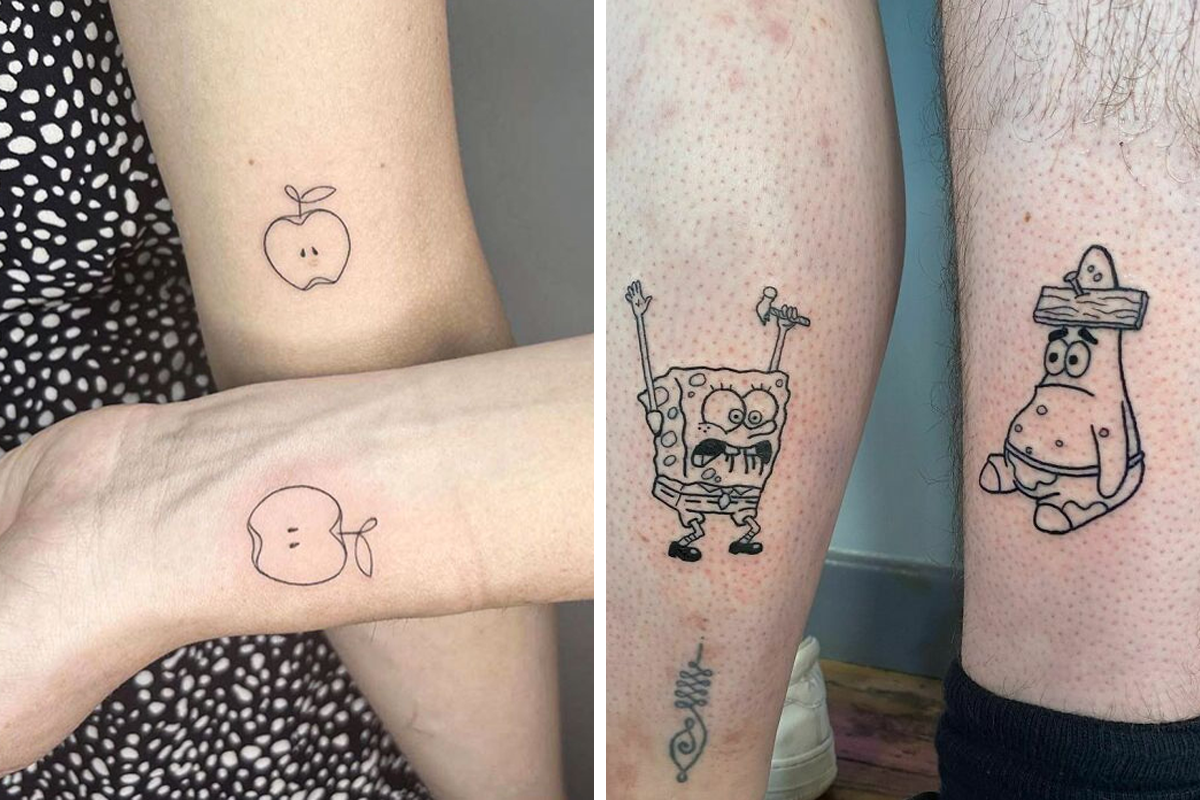The image consists of two side-by-side panels showcasing matching tattoos on different body parts. The left panel features two people standing shoulder-to-shoulder. One person's left arm, hanging down by their side, displays a simple black outline of an apple complete with two seeds, a stem, and two leaves. The second person's forearm is seen crossing the picture with an identical apple tattoo. In the right panel, there are two separate legs each adorned with a tattoo above the ankle. One leg has an outline of SpongeBob SquarePants accompanied by a squiggly music note underneath, while the other leg showcases a tattoo of Patrick Star. The tattoos in both panels are uniformly black outlines, contributing to a whimsical, coordinated display of body art that uses different parts of the body to portray complementary designs.